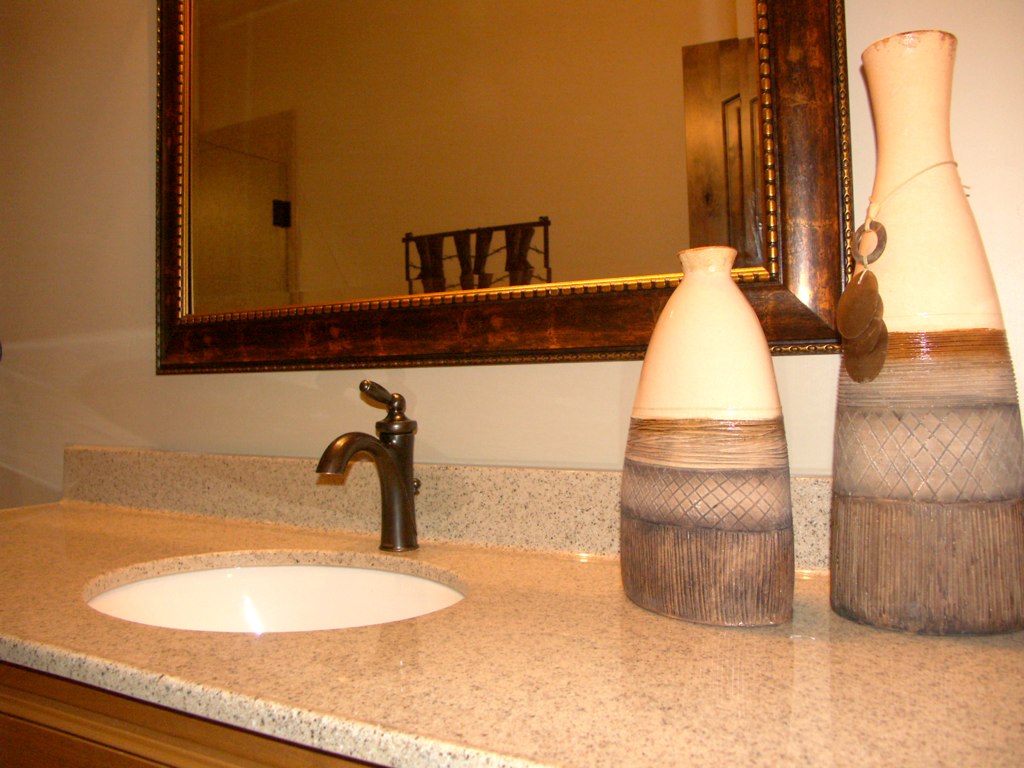This image captures the intimate setting of a bathroom, bathed in a warm yellow-orange glow likely emanating from the lightbulb in the room. In the foreground, a marble-style countertop is adorned with a small, circular sink. The sink is equipped with a dark, dull silver mixer tap that features a round, curved spout. Below the countertop, a teak-colored cabinet peeks out, hinting at its functionality and adding a rustic charm.

Behind the sink stands a mirror with a dark brown, intricately patterned frame, with hints of reddish-brown highlights that lend it an antique appearance. The mirror reflects a partially open door and an indistinct object, adding an element of curiosity to the scene.

To the right of the sink, two art pottery vases add an artistic flair. These vases share the same pattern but differ in size; the shorter one has a smaller opening while the taller one boasts a wider spout. The taller vase is also adorned with a string and pendant, giving it an extra touch of character. Both vases feature four distinct patterned sections: the bottommost section has vertical lines encircling the vase, above it lies a criss-cross pattern, followed by a ring of concentric horizontal lines, and finally, the upper halves of the vases are plain white. The lower three sections share a cohesive brown color scheme, which juxtaposes elegantly against the white upper half. 

This detailed setup, from the color tone and light source to the intricate details of the vases, creates a harmonious and inviting bathroom atmosphere.